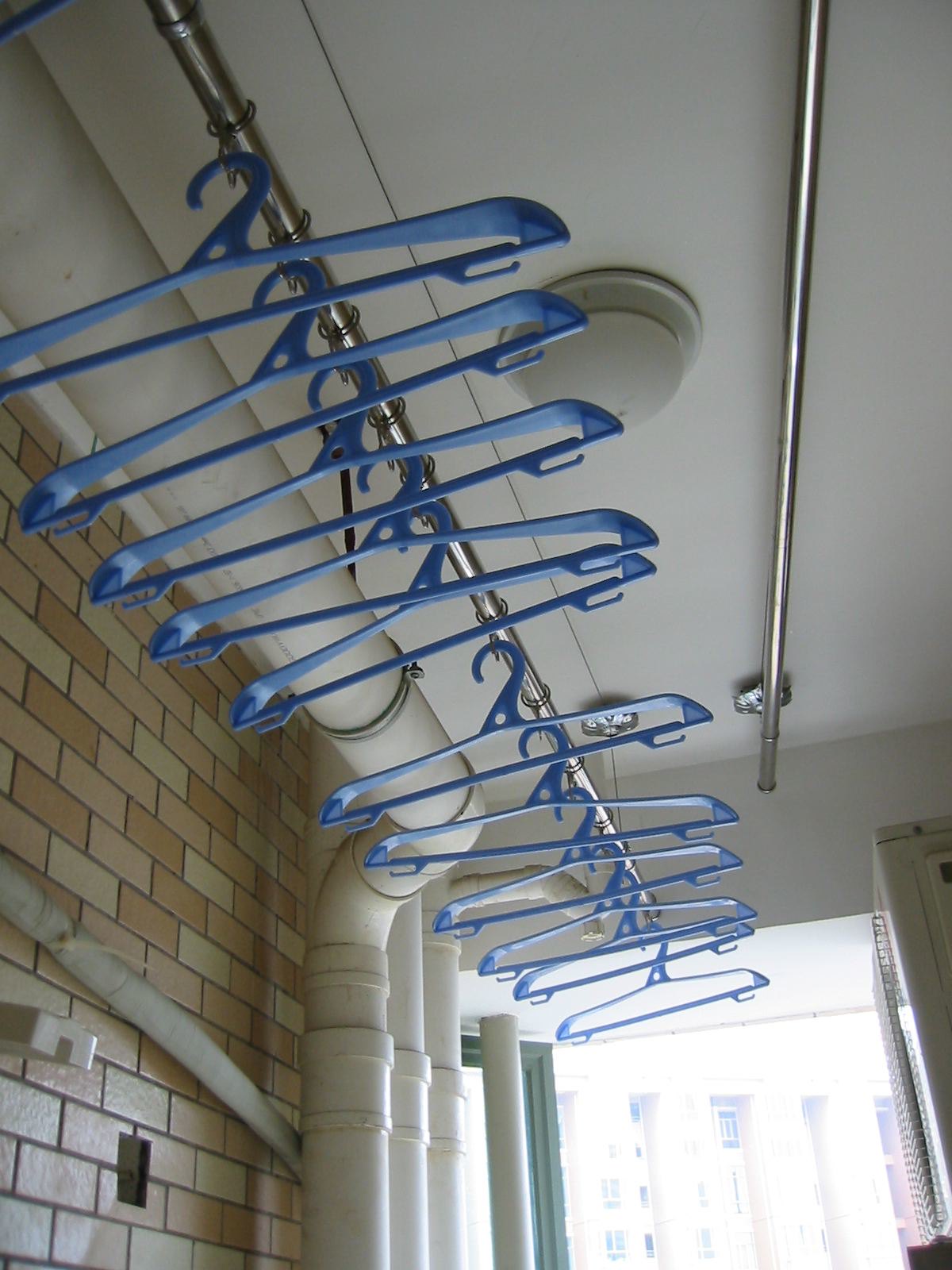This color photograph captures an upward view of the corner of a building's interior, possibly a dry cleaner's store. The image prominently features thick, white water pipes running vertically along a corner with tiles in shades of brown, light brown, and dark beige. From the ceiling hang two parallel chrome-plated rods, with one holding approximately eleven blue plastic coat hangers. These rods are secured by fixtures at their ends. The scene includes an open window in the background, through which bright sunlight illuminates a building outside. The overall setting is accentuated by a light fixture with a solid white glass dome positioned centrally on the ceiling.